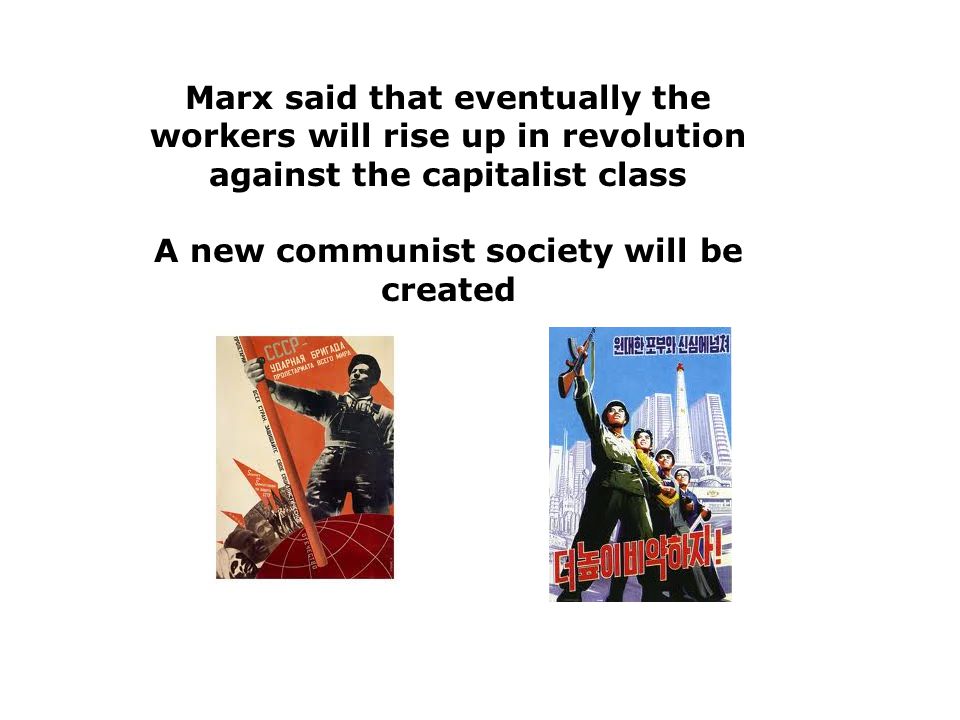The image features a predominantly white background with a prominent caption in bold, black Tahoma font at the top. The caption, positioned centrally, reads: "Marx said that eventually the workers will rise up in revolution against the capitalist class. A new communist society will be created." Below this text, the image is divided into two distinct sections featuring smaller pictures.

On the lower left, there is a rectangular image resembling a book cover. It depicts a black and white figure of a man holding an orange pole extending over a maroon, spherical globe shape. Above the man's head, the text "CCCP" is written, and additional words in a different language are inscribed below. The color scheme includes shades of orange, red, and gray.

The lower right section of the image shows a group of four people, likely soldiers, standing against a backdrop of white buildings and a blue sky. The person in the front holds a rifle, while the others seem to be looking upward. They are dressed in green uniforms. Red text in a foreign language is positioned across the bodies of the individuals and over the cityscape behind them.

These images combine visual elements and text to convey strong communist propaganda themes.